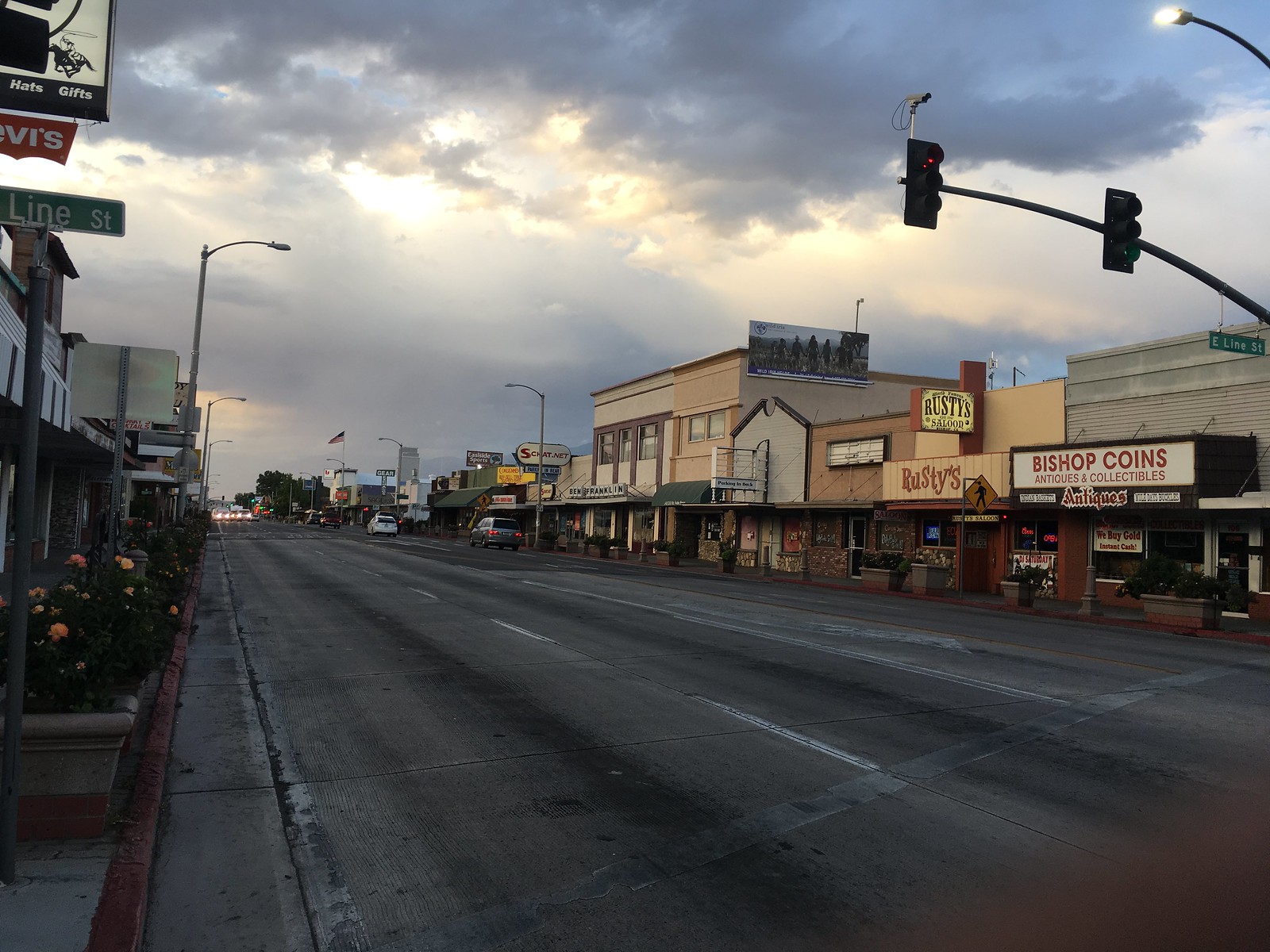The image depicts a gloomy sky dominated by gray clouds with faint rays of light breaking through. On the left side, there is a white structure with a red sign that reads "Hatskiss Levi." Below that, a street sign reads "Lions Creek." The road beneath is gray with white lane markings, leading into the distance where it becomes noticeably darker. 

In the background, several cars are parked along the street. To the far left, colorful flowers add a splash of contrast to the scene. The right side of the image features numerous buildings, some adorned with wood paneling and billboards. One prominent billboard displays the name "Rust-Eze" in bold red letters. Another sign reads "Bishop Coins, Antiques, and Collectibles."

Traffic lights are present on both sides of the street, though their signals are not illuminated. A street lamp stands nearby, adding to the urban atmosphere. The name "Mr. Rusilatov" appears in the context, possibly indicating a business or individual related to the scene.